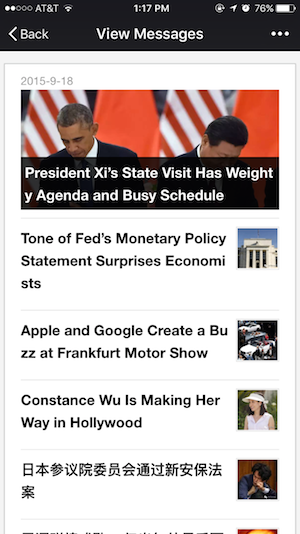In this multifaceted image, various elements converge to paint a detailed and vibrant scene. At the center, President Xi Jinping and former President Barack Obama are prominently featured, standing with 2 American flags and 2 Chinese flags behind them, symbolizing a state visit. Both leaders appear engaged, underscoring a busy agenda and tight schedule. The backdrop includes a white building, likely indicative of a significant governmental or historical site.

Overlaying the image are multiple icons and text snippets, enhancing the context further. On the top left, there are notifications including "AT&T Wi-Fi 117," an "alarm clock," and a "76% battery" symbol. Nearby, an arrow, circles, and dots in black and white also appear, possibly indicating interactive elements or design features.

In the mix are headline snippets that bring additional layers to the narrative. "Tone of Fed's Monetary Policy Statement surprises economists" and "Apple and Google create a buzz at Frankfurt Motor Show" highlight significant economic and technological developments. Another snippet, "Constance Wu is making her way in Hollywood," brings a cultural touch to the image. A woman in a white shirt and white hat stands next to a man with black hair, adding a personal, human aspect to the visual story. Meanwhile, Chinese symbols are also included, paying homage to the international dimension of Xi’s visit.

A golf cart is subtly placed within the scene, perhaps indicating the scale and accessibility of the venue or event. Overall, the intricate collage of images, text, and symbols encapsulates a bustling environment rich with political, economic, and cultural significance.